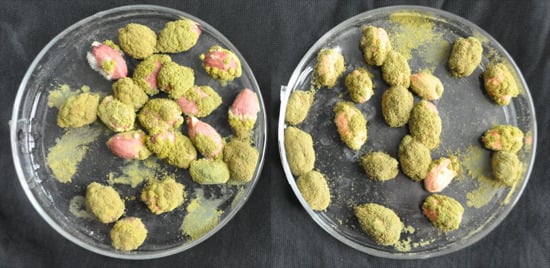The image depicts two clear Petri dishes, placed side-by-side against a nearly black background. Each dish contains approximately 20 small, roundish objects. These objects appear to be buds or nuts, some of which are pink, while most are covered in a green, mossy, fuzzy substance that leaves a powdery residue on the dishes. The dish on the left has more visible pink buds compared to the one on the right, where only one bud shows a significant amount of its original pink color. The green fuzziness can be seen smudged around both dishes, indicating that it comes off easily. The objects in the dish on the right are slightly more spread out compared to those in the dish on the left.